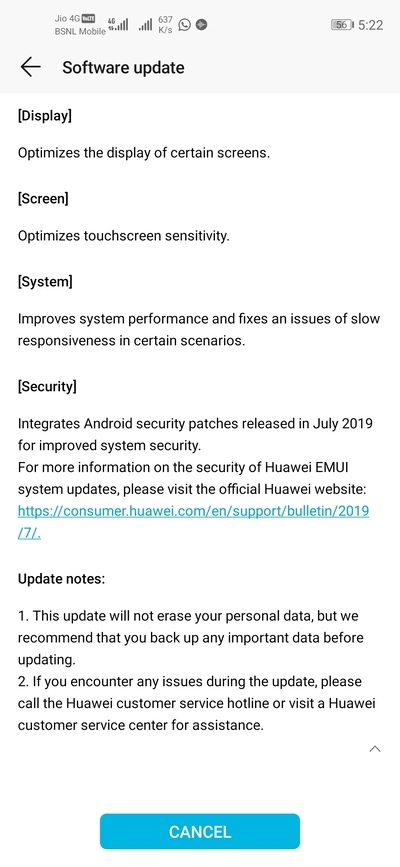A detailed image caption for the provided scenario could be:

"A photograph taken from a smartphone displays a software update screen. The top section of the screen is shaded gray, indicating the 'Software Update' title, which is accompanied by a left-pointing arrow icon on the left side. Below this section, the background is predominantly white. The screen text is displayed in black print and details various aspects of the update:

- 'Display' section mentions that it 'optimizes the display of certain screens.'
- 'Screen' section notes that it 'optimizes touchscreen sensitivity.'
- 'System' section specifies that it 'improves system performance and fixes an issue of slow responsiveness in certain scenarios.'
- 'Security' section highlights that it 'integrates Android security patches released in July 2019 for improved system security.'

A teal-colored hyperlink provides more information about the security of Huawei EMUI system updates, directing users to the official website. Further down, 'Update Notes' reassure users that 'this update will not erase your personal data, but it is recommended to back up any important data before updating.' Additional information follows, listed as point number two. At the bottom of the screen, there is a teal 'Cancel' button."